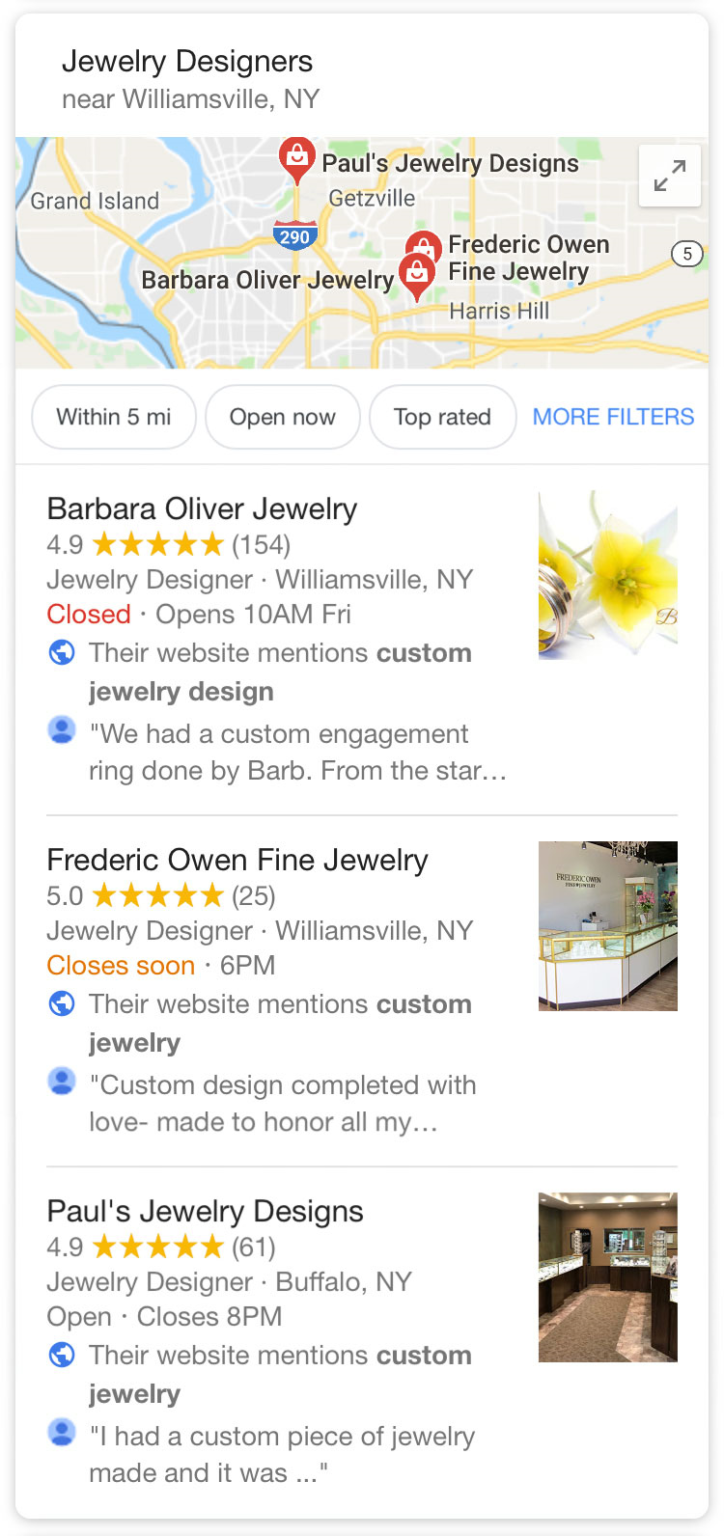Screenshot of a jewelry-related search conducted on a smartphone near Williamsville, New York. At the top of the screen, the search query "jewelry designers" is prominently displayed on a white banner with bold black text. Below the search bar, in gray text, it indicates the location "near Williamsville, New York." A small map highlights three jewelry stores: Barbara Oliver Jewelry, Frederick Owen Fine Jewelry, and Paul's Jewelry Designs.

Additionally, several filters have been applied to the search results: stores within five miles, currently open, and top-rated options, among others. 

1. **Barbara Oliver Jewelry**: Rated 4.9 stars based on 154 reviews. The store is currently closed and will reopen at 10 a.m. on Friday. It specializes in custom jewelry design, as noted by a nearby review icon featuring a flower.

2. **Frederick Owen Fine Jewelry**: Holds a 4.0 star rating from 25 reviews and is also closed, with operating hours until 6 p.m. Their website mentions a focus on custom jewelry, accompanied by a review icon displaying an image of a jewel case.

3. **Paul's Jewelry Designs**: This store has a 4.9 star rating from 61 reviews. It remains open until 8 p.m. and offers custom jewelry services, with a review icon showing the interior of the store.

Each listed store includes ratings, reviews, and specific details about their custom jewelry services.